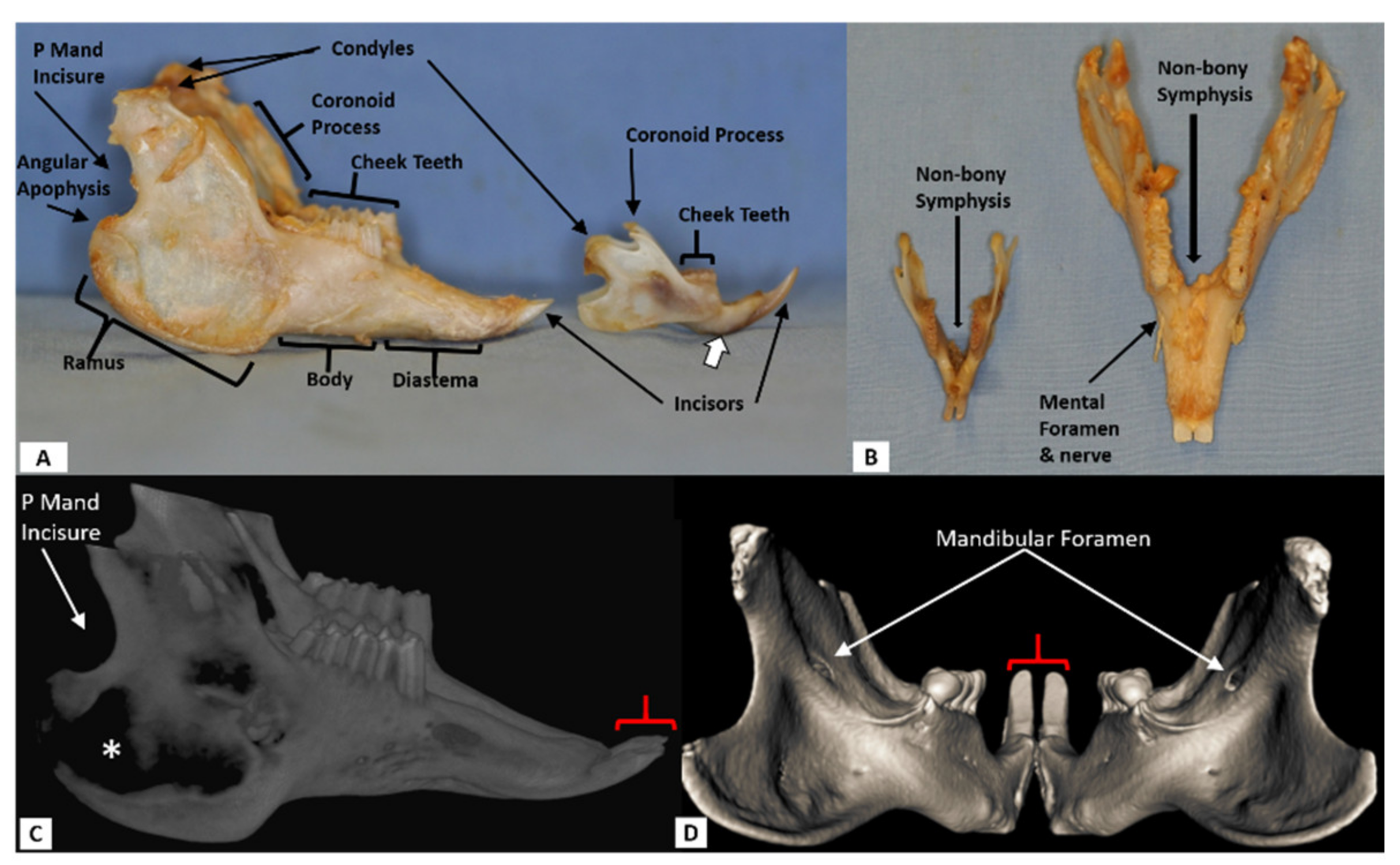The image shows a detailed diagram of the skeletal structure of a creature, focusing primarily on the dental and mandibular regions. The top sections display labeled illustrations of the structure, which includes the cheek teeth, body, diastema, incisors, ramus, angular apophysis, condyles, and coronoid process. The labels on the top left identify the P-Man incisor, while arrows point to features such as the non-bony symphysis and the mental foramen and nerve on the right. The bottom sections provide additional diagrams and labelings, with sections marked C and D highlighting the P-Man incisor and the mandibular foramen using red marks. The bottom right features x-ray renderings of the structure, providing a different view of the same labeled elements. The teeth appear yellowish in color, adding to the detailed depiction of the bones and teeth in various perspectives. This composition effectively showcases the intricate features of the creature's skeletal and dental anatomy.